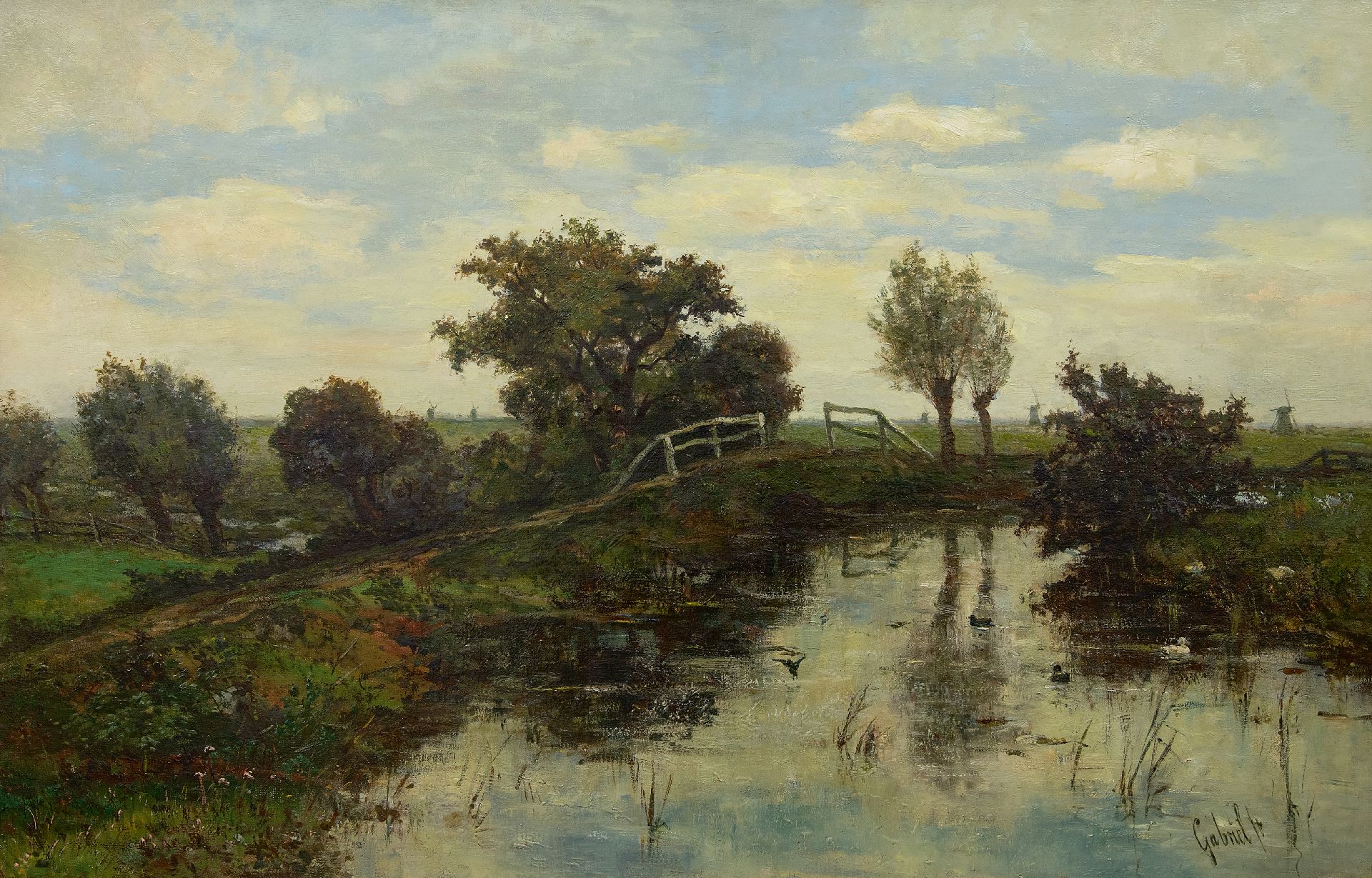The image is a detailed oil painting that depicts a bucolic yet dimly lit country scene, possibly resembling the works of John Constable. The painting is signed by an artist named Gabriel. In the foreground, a pond reflects a sky partially covered in white clouds and pale blue patches. The pond has water vegetation and thin weeds peeking out. Encircling the pond is a mix of green, reddish, and brown grass, alongside a small brown road with sections having a white fence. 

On the left of the scene, the road slightly slopes down a hill towards a green field dotted with trees and a wooden fence. Directly in front, a large tree stands tall, while slightly to the right, a leafless tree adds a stark contrast. A partially completed or railed bridge spans a section of the water, leading into the distance. To the right, a bush marks the edge of the riverbank, which curves gently towards the background.

In the distance, the landscape reveals more green fields and small, gray-colored windmills, hinting at a Dutch countryside. The trees beyond the road have brown trunks and varying foliage, with one tree notably bearing white-looking foliage, creating a subtle focal point amidst the verdant surroundings.